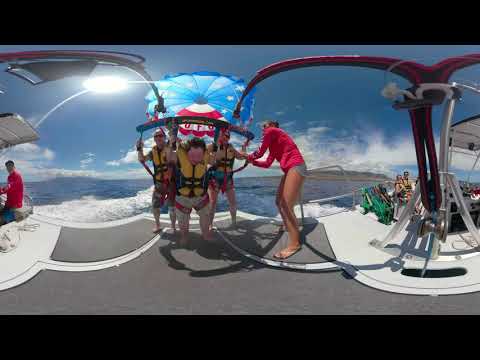This is a panoramic and somewhat distorted, exterior, color, daylight photograph of a group of people preparing for a parasailing adventure on a boat. The image is bordered by thick black rectangles at the top and bottom, indicating it may have been captured from a video. In the mid-ground, three individuals, dressed in swim trunks, shirts, and bright yellow life preservers, are harnessed to a glider with an American flag-patterned parachute, featuring red, white, and blue colors. A woman in a long-sleeve pink shirt, very short shorts, and sandals is ensuring that their harnesses are secure. The boat's flat, gray surface with a protective metal railing is visible beneath the group, and a large wake trails behind the boat in the ocean. Additional individuals in yellow life vests are seated on the right side of the boat. The sky is mostly blue with scattered white clouds, and the sun is shining brightly. Land is faintly visible in the distance to the back right.